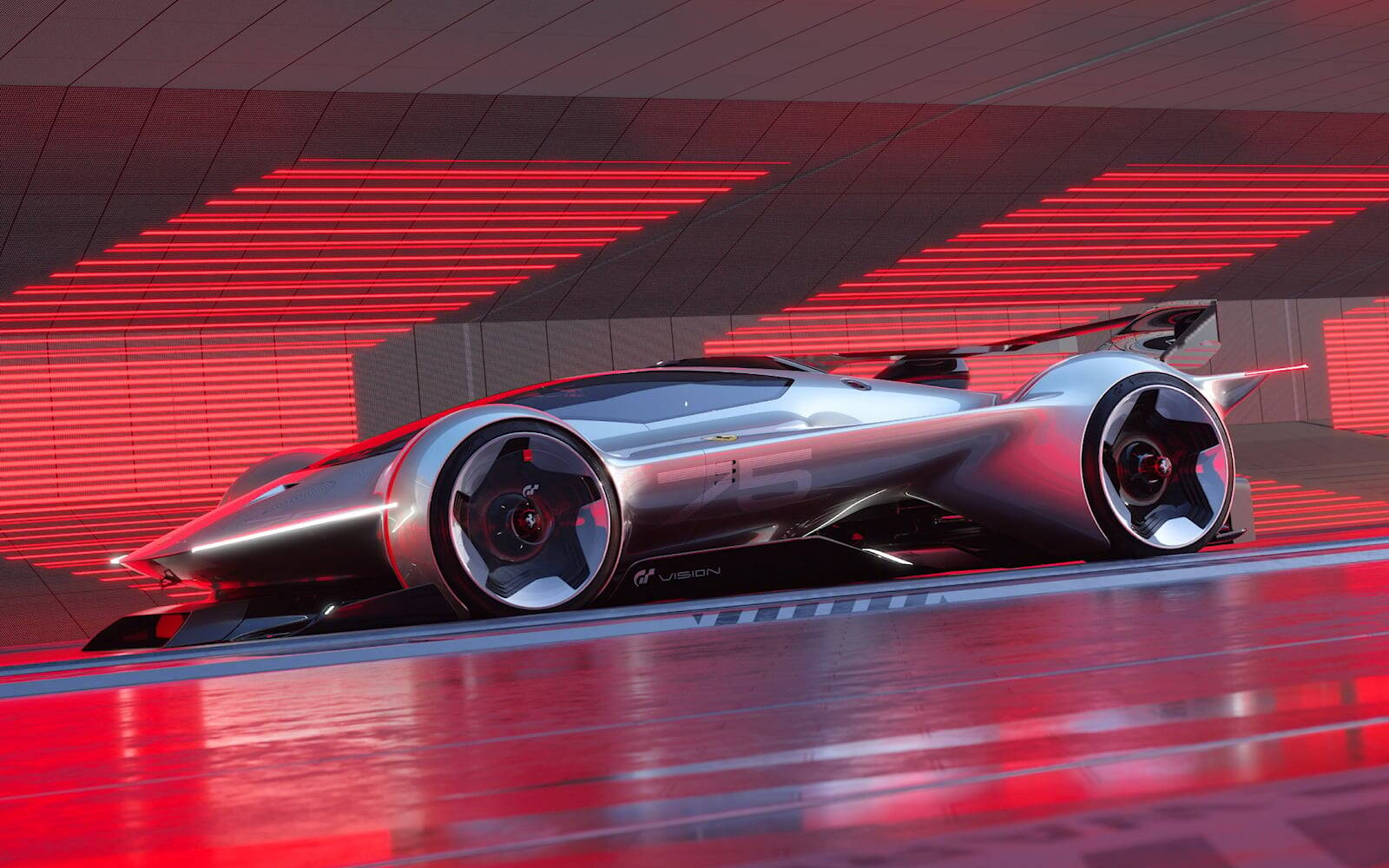The image depicts a highly futuristic and sleek silver sports car situated in a possibly indoor showroom. The car stands out with its shiny, smooth body and pointed, sharp features giving it a modernistic flair. One of the car's most striking aspects is its rounded, smooth metal wheels, which are encased within the car's body, differing from traditional car designs. A prominent, blacked-out windshield adds to the car's high-tech appearance. The setting features a maroon backdrop with dark lines and vibrant horizontal red lines running from the top to the bottom of the image. These red lights reflect on the shiny, slightly silver ground, creating a sophisticated ambiance. Below the car, a black panel with the word "Vision" is inscribed in white letters, further emphasizing the advanced nature of the car. Notably, no doors are visible, adding to the car's mysterious and avant-garde design.